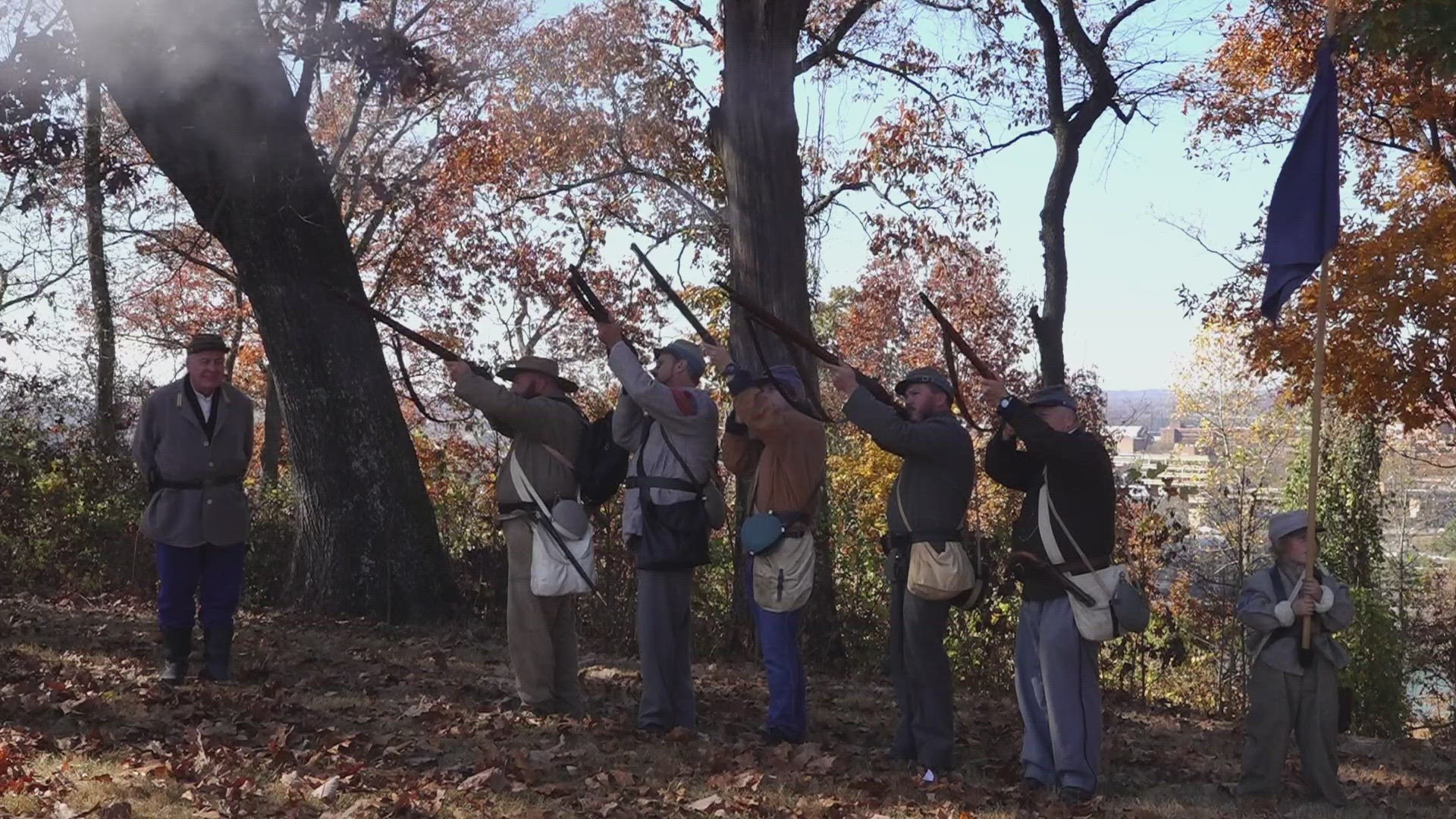In this vibrant autumn scene, an authentic Revolutionary War reenactment unfolds on a hilltop overlooking a city skyline, which glimmers under a bright blue sky. Brown and golden leaves, both scattered on the ground and clinging to the trees, create a picturesque fall backdrop. At the center, five men stand aligned, dressed in traditional Revolutionary War attire—long shirts cinched by belts, trousers, and cross-body satchels. They brandish long rifles, pointing them skyward in unison. Beside them is an older figure, seemingly a leader or general, distinguishable by his unique hat and buttoned outfit. On the right, a small child clutches a blue flag, adding to the historical ambiance of the scene. The reenactors' detailed costumes and the natural surroundings evoke a rich sense of history and seasonality.